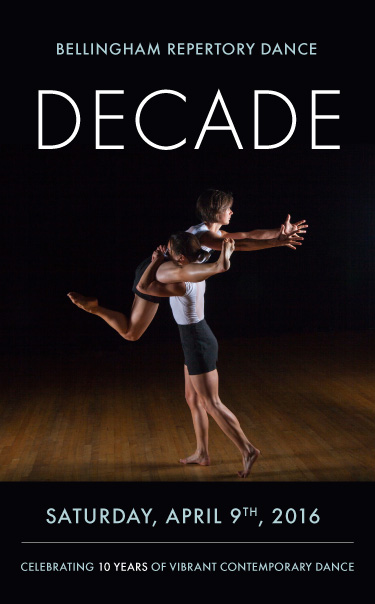The poster for the event features Bellingham Repertory Dance in large white letters at the top, followed by the title "Decade". Below, the date "Saturday, April 9th, 2016" is prominently displayed above a thin line of text that reads "Celebrating 10 Years of Vibrant Contemporary Dance." The background is predominantly black, emphasizing the central image of the poster. In the middle, two women are captured in a dynamic dance pose on a wooden floor that fades into the black background. Both women are barefoot and dressed in black shorts and white tops. The woman on the bottom, standing on her toes of one foot while the other foot is flat, gracefully lifts the other woman over her shoulder. The lifted woman has her arms and legs outstretched, creating a striking visual of balance and movement. Both performers are Caucasian with short hair; the woman lifting has a ponytail, while the one being lifted has a bob cut. The composition and details of the poster vividly convey the celebratory and artistic spirit of the event.